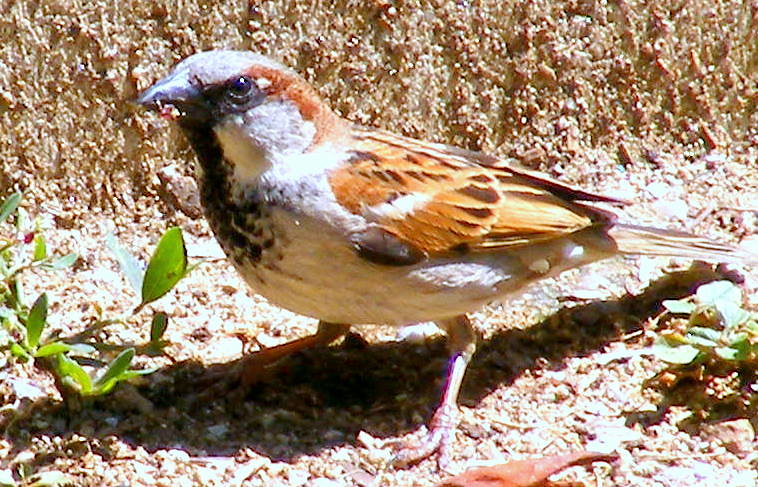This close-up image captures a small bird standing on a dirt ground. The bird has a white belly, a white neck that extends to its head, and white cheek feathers. Its back is adorned with orange and brown feathers, while its head and wing feathers also feature shades of orange, brown, and red. The bird's throat and front chest are marked with black feathers, accentuating its black beak, which is holding either a small flower or a tiny worm.

The setting is outdoors during the daytime, with high lighting that casts a shadow beneath the bird. Surrounding the bird, there are a few small green plants with visible green leaves and some scattered twigs near its feet. The background features what appears to be a small dirt wall or possibly a stucco wall, adding to the earthen setting. Despite the detailed glimpse of the bird, the image is somewhat blurry and grainy. The bird stands in an active stance, looking away toward the camera.